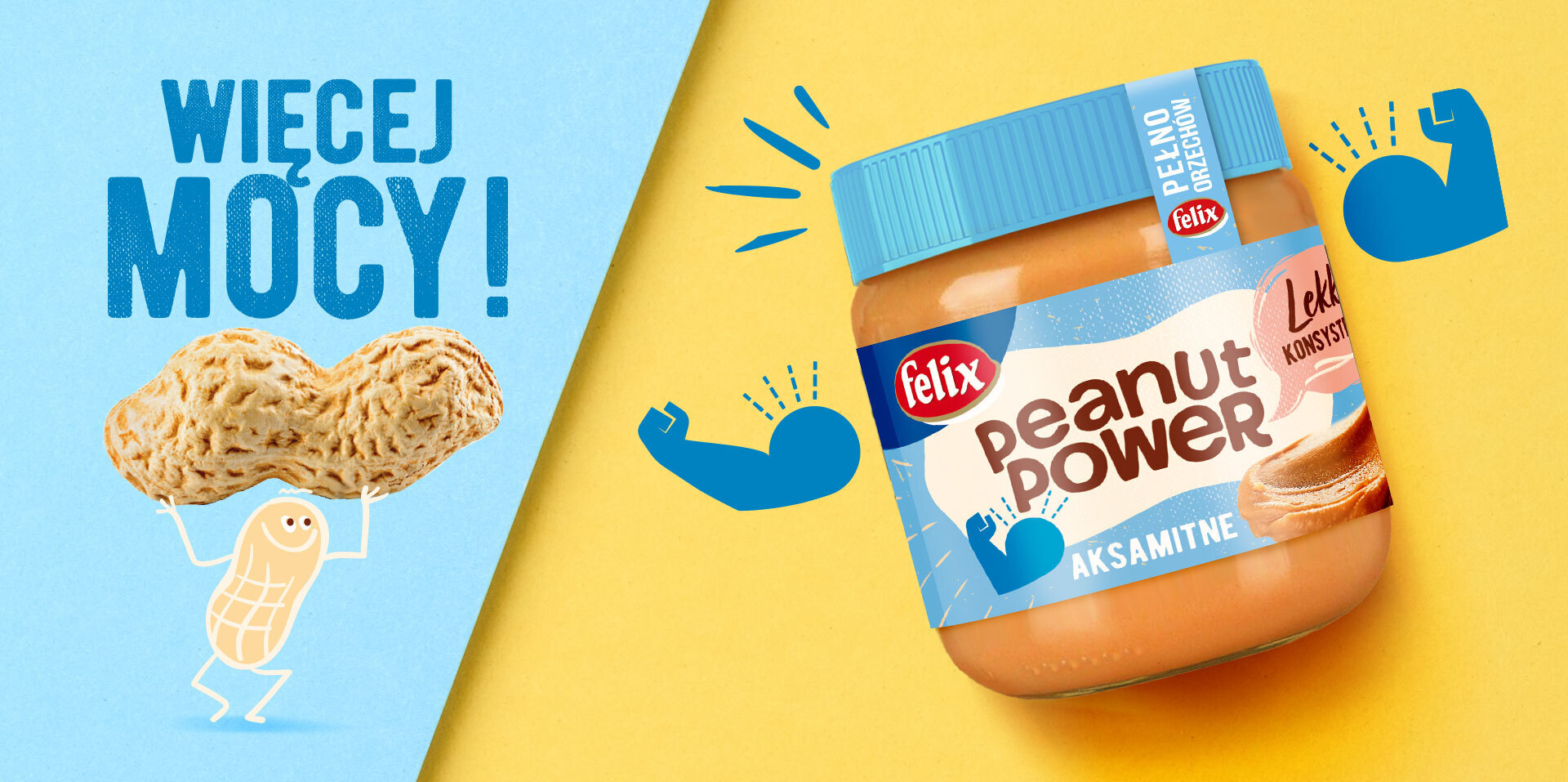This advertisement for Felix's Peanut Power peanut butter features bold and vibrant colors, primarily yellow and light blue. On the left side of the advertisement, set against a blue background, there's a cartoon peanut character with limbs, smiling and looking to the right while holding a large peanut above its head. The text above the character is dark blue and says something like "Weseej Mosey." In the center, a prominently placed Felix Peanut Power jar with a light blue screw-on lid takes center stage. The jar’s label is light blue with a white peanut-shaped area in the middle, where "Peanut Power" is written in brown text. Above this, the brand name "Felix" is displayed in a red oval logo, though somewhat obscured, it might include extra details such as "L-E-K-K" in a salmon speech bubble. Flanking the jar on both sides are illustrations of muscular arms, rendering the jar with a sense of strength and vigor, visually emphasizing how this peanut butter will build strong muscles.